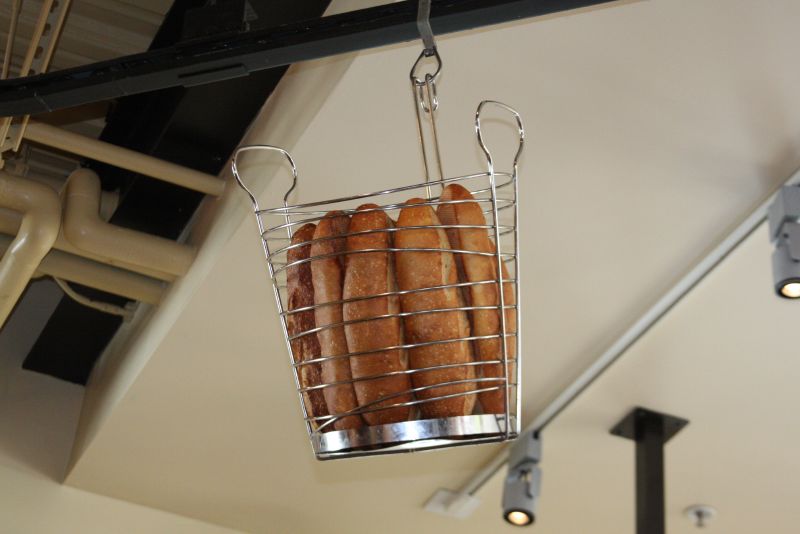This is a detailed color photograph taken from an upward-facing angle, likely in a restaurant or kitchen setting. Dominating the center of the image is a wire basket, cylindrical in shape with horizontal silver wire hoops forming its sides and vertical wires creating handles on either side. The basket is suspended by a hook from a black rod affixed to the ceiling. Within the basket are several vertically standing loaves of bread or pastries, their golden-brown tones sharply contrasted against the blurred background. To the lower right, gray track lighting can be seen running diagonally across the ceiling, accompanied by a black pole rising from the bottom corner of the image. The upper left reveals light yellow insulated pipes, contributing to the industrial aesthetic of the space. A black beam also traverses the image, adding to the structural complexity of the ceiling. The image's focal point remains the intricately detailed basket of bread, set against a backdrop of subtly blurred ceiling fixtures and industrial elements.